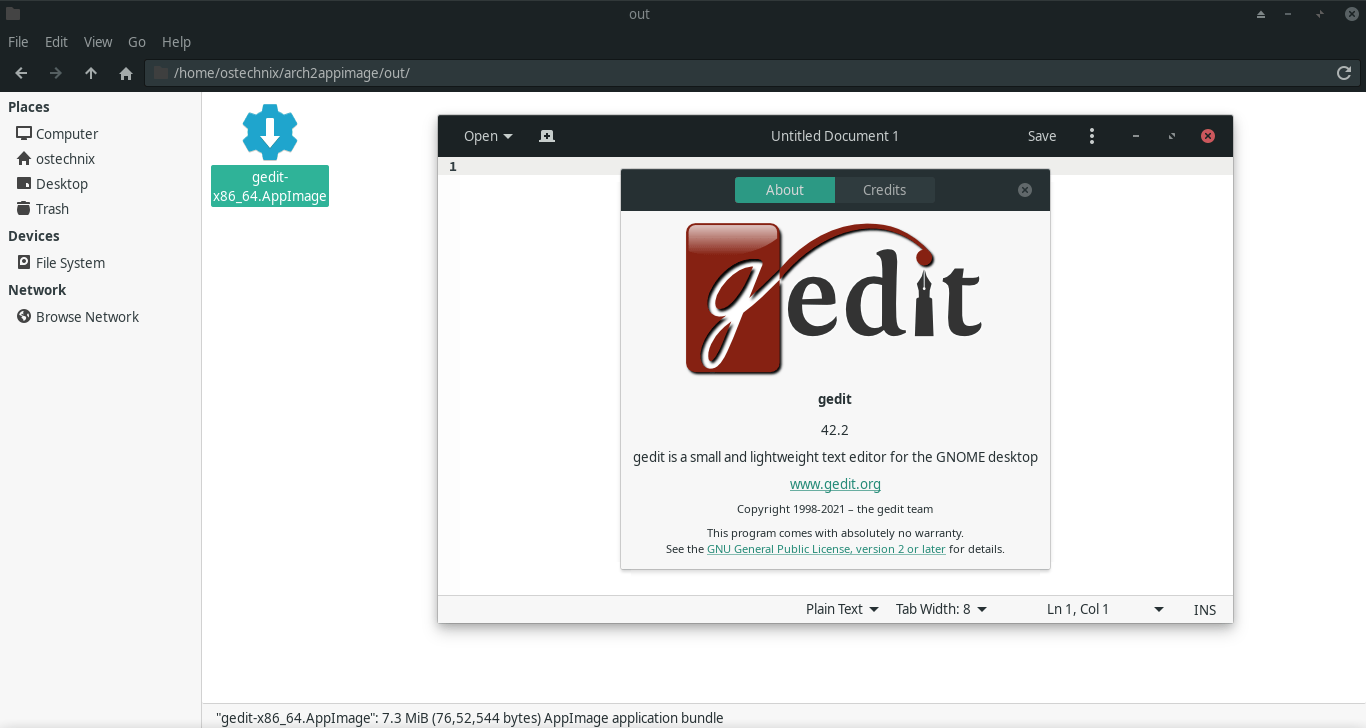The image features a user interface layout with several distinct elements. At the top, there is a long black rectangle housing a search bar. Directly below this, on the left side, is a section labeled "Places," in black text, accompanied by several icons:

- A black square icon labeled "Computer"
- A black square with a white dot icon labeled "Desktop"
- A small black square icon labeled "Trash"

Further down, there are categories listed:

- "Devices"
- "File System"
- "Network"

Beneath the "Network" category, a black circle option labeled "Browse Network" is available.

On the right side of the interface, there is a blue settings wheel with a white downward-pointing arrow. The arrow indicates the direction toward a green rectangle containing some white text.

In the central area, the main focal point of the image is an untitled document. Below, a green rectangle displays the word "About," flanked by the word "Credits." Additionally, there is a distinctive lowercase "g," half white and half burgundy. This "g" is enclosed in a burgundy-colored square box. Finally, to the right of the "g" is the word "Edit," marking the end of the information displayed in the image.